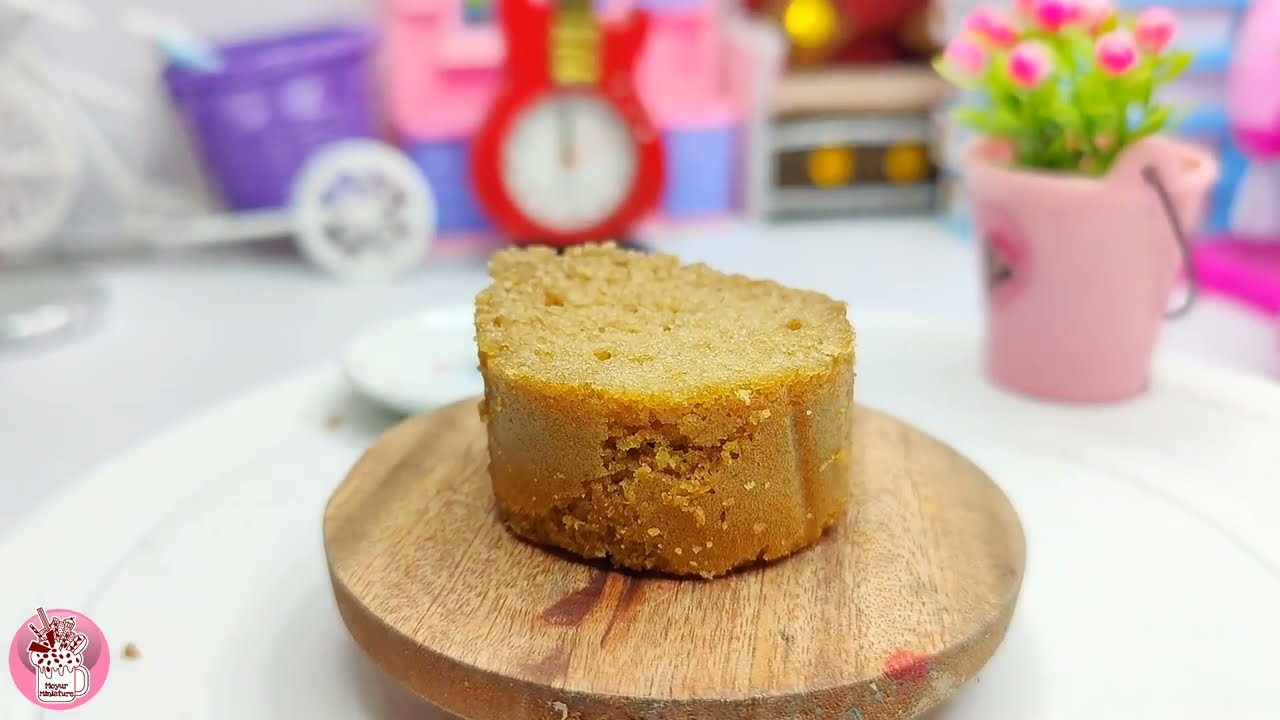In the foreground of this horizontal rectangular image, a slice of golden-brown pound cake rests on a round wooden tray with a light brown hue. The tray itself sits atop a larger white plate. The scene is vibrant with colors, featuring various items in the background, although they are blurred. Notably, there's a small pink bucket filled with green leaves and dark pink flowers on the right. To the upper left, a grayish-purple bucket is positioned next to a partially visible red and white toy guitar. The toys also include what looks like a purple stroller, a purple basket attached to a tricycle, and potentially other children’s toys, signifying a playful background that resembles a kid's room or playroom. The bottom left corner of the image features a tiny circular logo, white and pink in color, although the text is too small to discern. This setting, vibrant and slightly whimsical, seems to be styled as an advertisement for a confectionery company showcasing their pound cake.